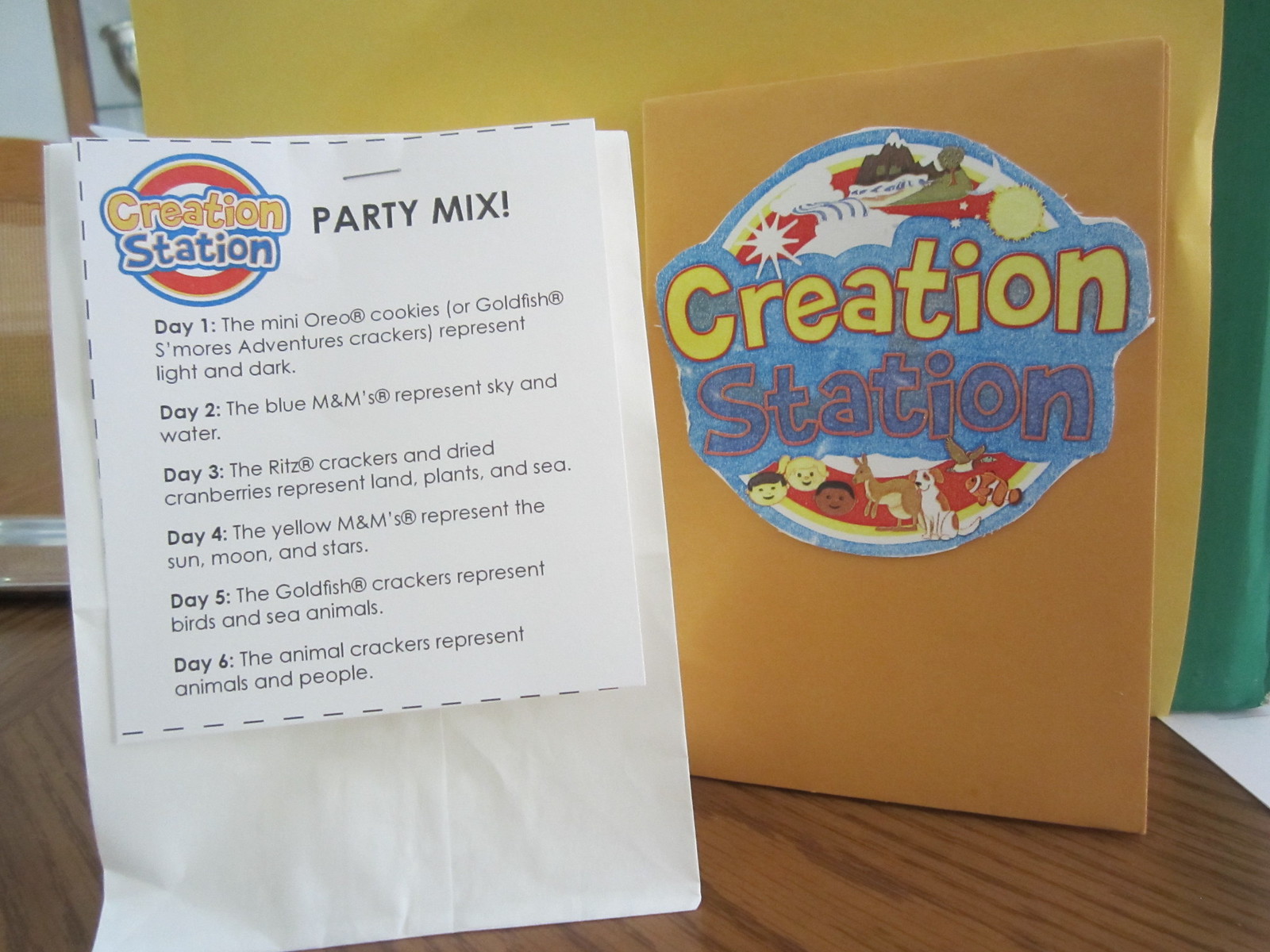The image depicts a sheet of paper with a small bag, both set on a wooden surface that could either be a table or floor. The paper, positioned centrally in the image and likely part of an indoor scene taken during daylight, is titled "Creation Station Party Mix" and features detailed instructions associated with various days:

- **Day One:** Mini Oreo cookies or Goldfish S'mores Adventure Crackers symbolize light and dark.
- **Day Two:** Blue M&M's represent the sky and water.
- **Day Three:** Ritz crackers and dried cranberries stand for land, plants, and sea.
- **Day Four:** Yellow M&M's represent the sun, moon, and stars.
- **Day Five:** Goldfish crackers signify birds and sea animals.
- **Day Six:** Animal crackers depict animals and people.

The sheet is adorned with a sticker that serves as a logo with illustrations of children, a dog, a fish, a sun, mountains, and trees. Additionally, accompanying text embellishes the yellow paper, enhancing the visual appeal with the "Creation Station" title and cartoon animals. The scene vividly showcases assorted colors like brown, white, red, blue, yellow, green, and orange.